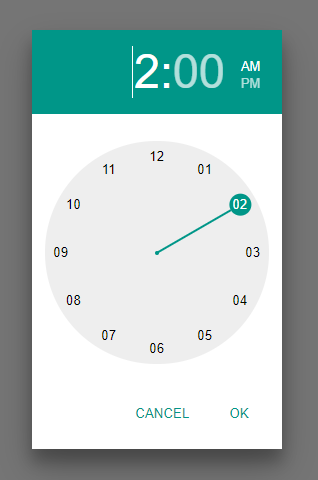A vertical, portrait-style image features a rectangular interface set against a medium gray background. The interface is divided into two distinct sections. At the top, a medium greenish-blue bar displays the current time setting, "2:00," in white text, with a thin vertical line adjacent on the left. To the right of the time, "AM" and "PM" options are presented, with "AM" highlighted in white to indicate its selection, while "PM" appears in a lighter gray shade.

Below this bar, the interface background shifts to white, showcasing a graphical representation of a clock. A light gray circle forms the clock's face, with numbers "01" through "12" arranged around its perimeter, mimicking a traditional clock layout. The number "02" is emphasized within a green box, from which a line extends to the clock's center, indicating the selected time of 2:00 AM. 

At the bottom of the interface, "Cancel" and "OK" options are presented in green text, providing control over confirming or discarding the time selection.